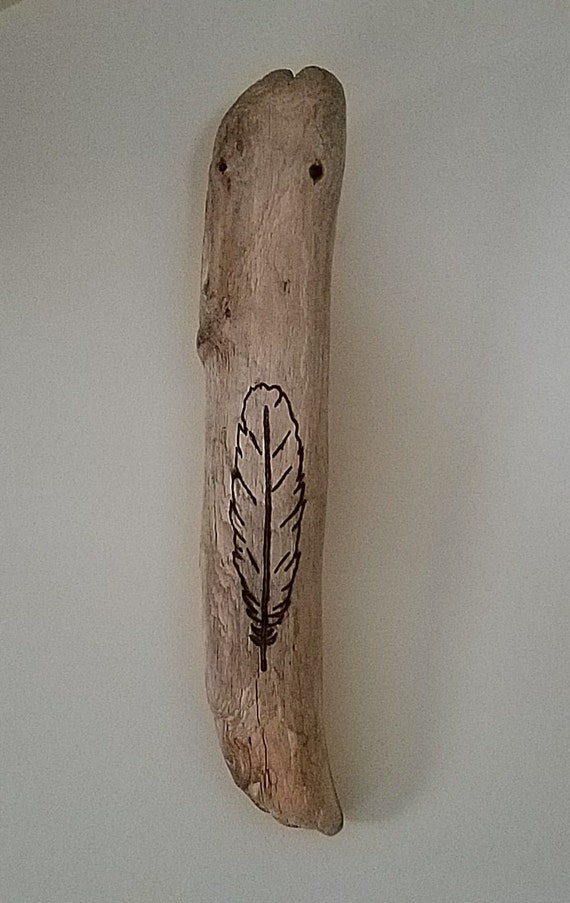Displayed against a gray background, this rectangular image features a carefully crafted piece of wood, resembling a thicker, arm-sized tree limb. The wood appears to be old and possibly fallen, minimally shaped and sanded to a smooth texture, suggesting a piece of pale-colored timber like beech, ash, or poplar. Dominating the focal point of the wood, just below the center, is a stylized feather, intricately rendered in black. This feather seems to have been either woodburned or painted onto the surface, standing out strikingly against the gray-beige hue of the limb. The work displays a high level of craftsmanship, making it suitable for display in a handmade Etsy store or even in a museum, although its primary function appears to be artistic rather than utilitarian.